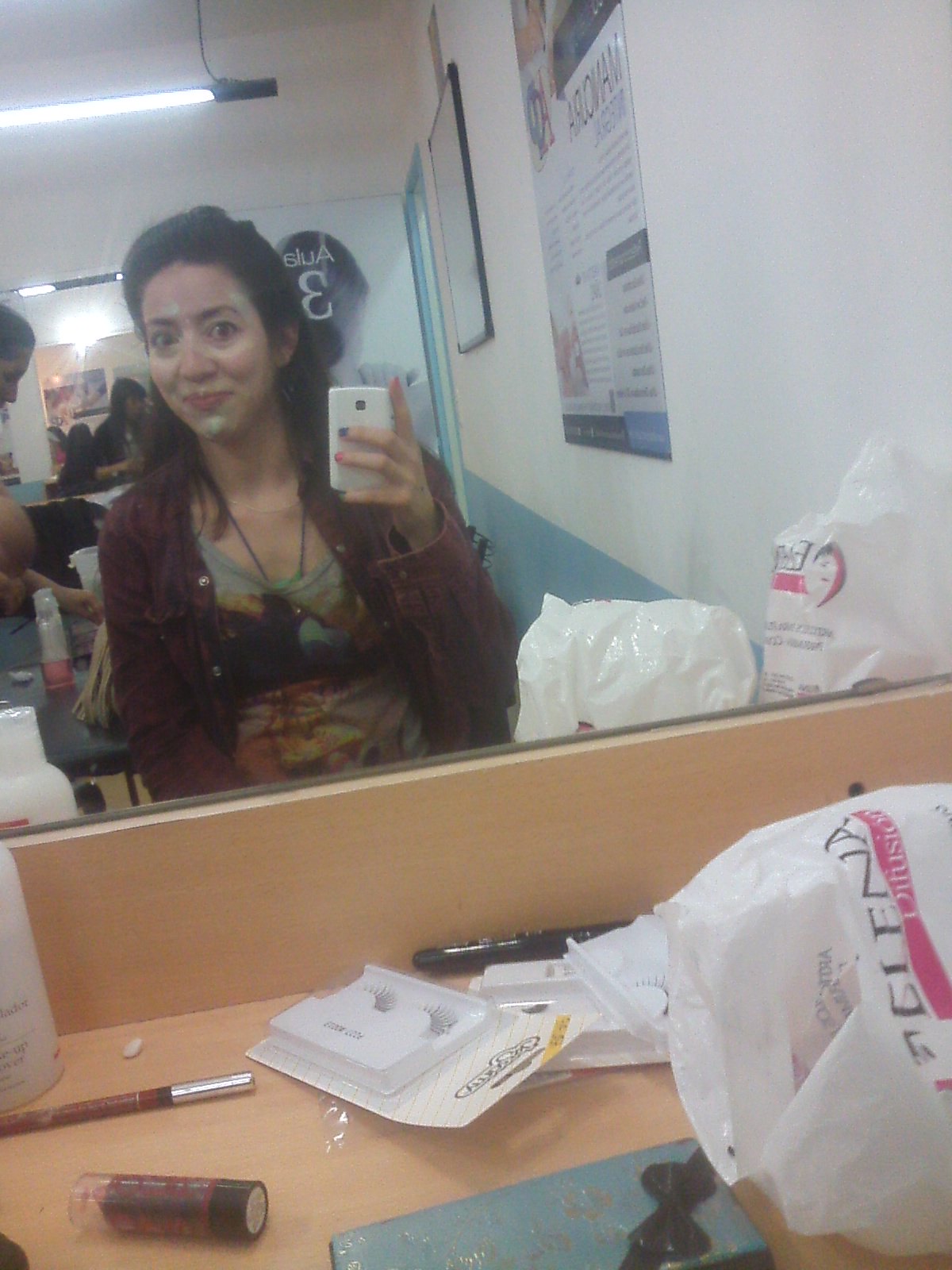This photograph captures a vibrant scene in a beauty salon, focusing on a woman in her late twenties or early thirties taking a humorous selfie in a mirror. Her long, dark hair is pulled back, revealing her pale, possibly Hispanic skin and pronounced cheekbones. She is wearing a distinctive brownish-reddish jacket over a colorful t-shirt with an abstract design featuring yellow, black, light blue, and grey hues. A blue necklace string peeks out from her t-shirt. 

The woman is holding a small, white phone in her right hand, capturing her reflection in the mirror. Her expression is playful, with a closed-lip smile suggesting amusement. Her dark, wide-open eyes emphasize her jovial mood. She has applied beauty cream in splotches on her chin, around her eyes, and between her eyebrows, adding a humorous touch to the image.

Behind her, the beauty salon buzzes with activity. Mirrors reflect various indistinct figures, and the walls are adorned with posters. A wooden counter beneath the mirror holds numerous beauty supplies like lipstick, eye shadow, and brushes, hinting at the cosmetic nature of the space. The overall scene is brightly lit by a large strip of light on the ceiling, and the walls are white with blue accents at the bottom.